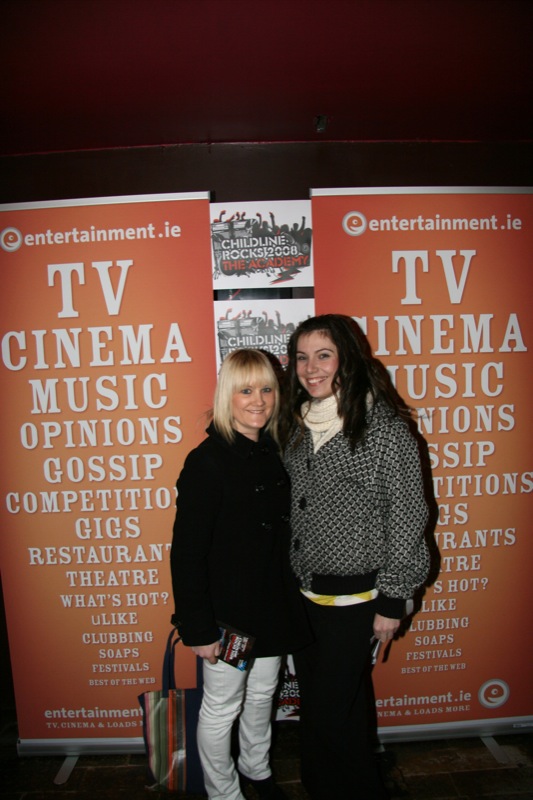In this detailed image, we see two individuals standing side-by-side in front of vibrant billboards with an orange background. The billboards prominently advertise "entertainment.ie," listing various categories such as TV, cinema, music, opinions, gossip, competition, gigs, restaurant, theater, what's hot, you like, clubbing, soaps, festivals, and best of the web. The text decreases in size from top to bottom and is predominantly white. Additional text within white squares states "Childline Rocks 2008," with "The Academy" appearing prominently as well.

The individual on the left is a shorter woman with brown hair accented by blonde sides and bangs. She is wearing a black suit jacket that reaches her hips and white pants. She holds a black booklet in one hand and has blue eyes, smiling brightly at the camera.

To her right stands a taller young girl with red, shoulder-length hair. She is also smiling widely and is dressed in a black and gray circle-patterned jacket with black buttons, a light white scarf, and black pants. Her hands rest just below her hips.

Both appear happy and are enjoying the moment, captured against the backdrop of these eye-catching advertisements.